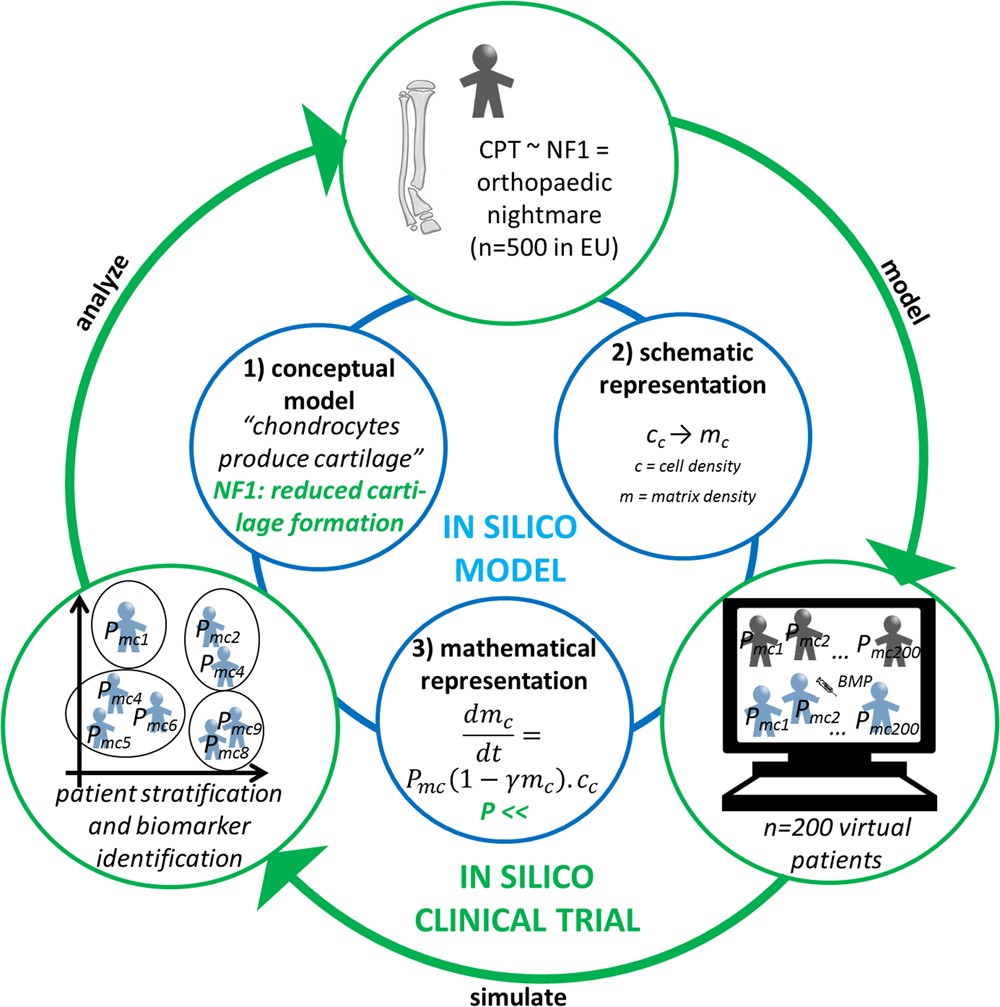The image depicts a detailed flowchart of a clinical trial process, primarily focused on orthopedic treatments. At the bottom, arrows form a full circle illustrating the cyclical nature of the trial. The stages begin with "Simulate," which encompasses patient stratification and biomarker identification. This is followed by "Analyze," featuring a leg bone, possibly indicating areas of orthopedic concerns (CPT, NF1, orthopedic). The next stage is "Model," showing a computer screen with virtual patients and mathematical representations of chondrocytes producing cartilage, along with factors like cell density and matrix density.

The outer circle represents the overarching trial phases, while the inner circle showcases a more detailed conceptual model with three blue sub-circles labeled as "Conceptual Model," "Schematic Representation," and "Mathematical Representation." This inner section is termed the "In Silico Model," emphasizing the virtual and computational aspects of the trial. The entire process highlights the integration of patient data, computational modeling, and the iterative nature of medical research in a clinical setting.